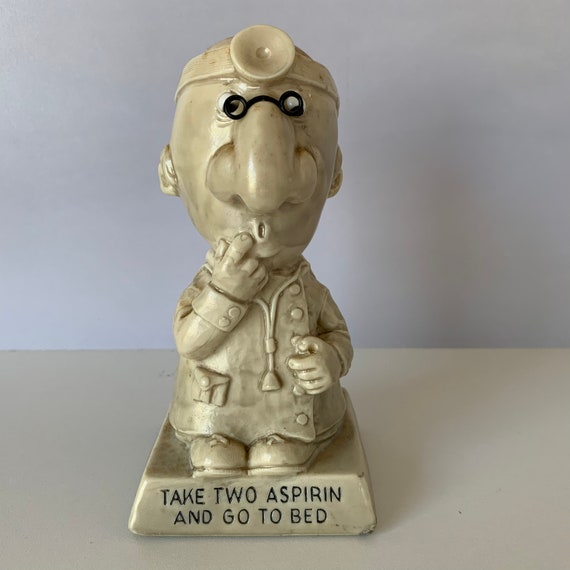This photograph, taken indoors against a light grayish blue wall, showcases a small, whimsical statue of a doctor. The 4-inch high and wide statue stands on an off-white countertop. The doctor, crafted from a plastic-heavy material with a slightly dirty ivory tone, dons a white coat, a stethoscope, old-fashioned spectacles, and a reflective headlamp. His caricatured face features exaggerated elements like a large nose, googly eyes, and a mouth shaped in an 'O', suggesting confusion or surprise, with his right finger resting against his lips. He sports oversized clown-like shoes, and his left hand is positioned at his waist. The base of the statue, engraved in black uppercase letters, bears the humorous text: "TAKE TWO ASPIRIN AND GO TO BED." This playful piece, with its detailed carving and off-white hues mixed with brown, captures a nostalgic, comic essence, reminiscent of something you might find in a dollar store.